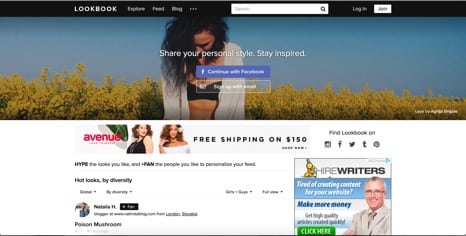Screen capture of an e-commerce website: 

**Header Section:**
- At the top of the page, there is a black navigation bar with blurred text that seems to read "Feed" and "Blog."
- On the top-left, a white book icon is present.
- Toward the top-right, there is a white search bar with a black magnifying glass icon. 
- Far right features a login option and a white button, likely labeled "Join."

**Banner Image:**
- Situated below the header, the banner spans horizontally from edge to edge.
- The banner showcases a scene with a blue sky and a treehouse in the background.
- In the center of the banner, a woman appears, wearing a black bra under a white sweater, with her head slightly tilted down.
- The overlaying text reads, "Share Your Personal Style, Stay Inspired."
- Below the message, there is a blue button prompting users to "Continue with Facebook" and another white button, though blurred, indicates a sign-in option, probably "Sign in with [another service]."

**Midsection:**
- On the top left of this section, the text "Avenue" appears next to a picture of two young women posing, likely models.
- Next to the photo, bold black lettering advertises, "Free Shipping on $150."
- On the far right, icons for Instagram, Facebook, Twitter, and Telegram are shown next to the phrase "Find Look Book on."

**Ad and Additional Text:**
- Beneath this, a generic Google ad is displayed, marked with an arrow in the upper right-hand corner and the text "Hire Writers."
- The left side text indicates that people are actively shopping, and refers to "Hot Looks by Diversity," although this is somewhat blurred and hard to decipher clearly.

Overall, the image captures various promotional elements, user action prompts, and social media connectivity options, framed within a clean, appealing layout.